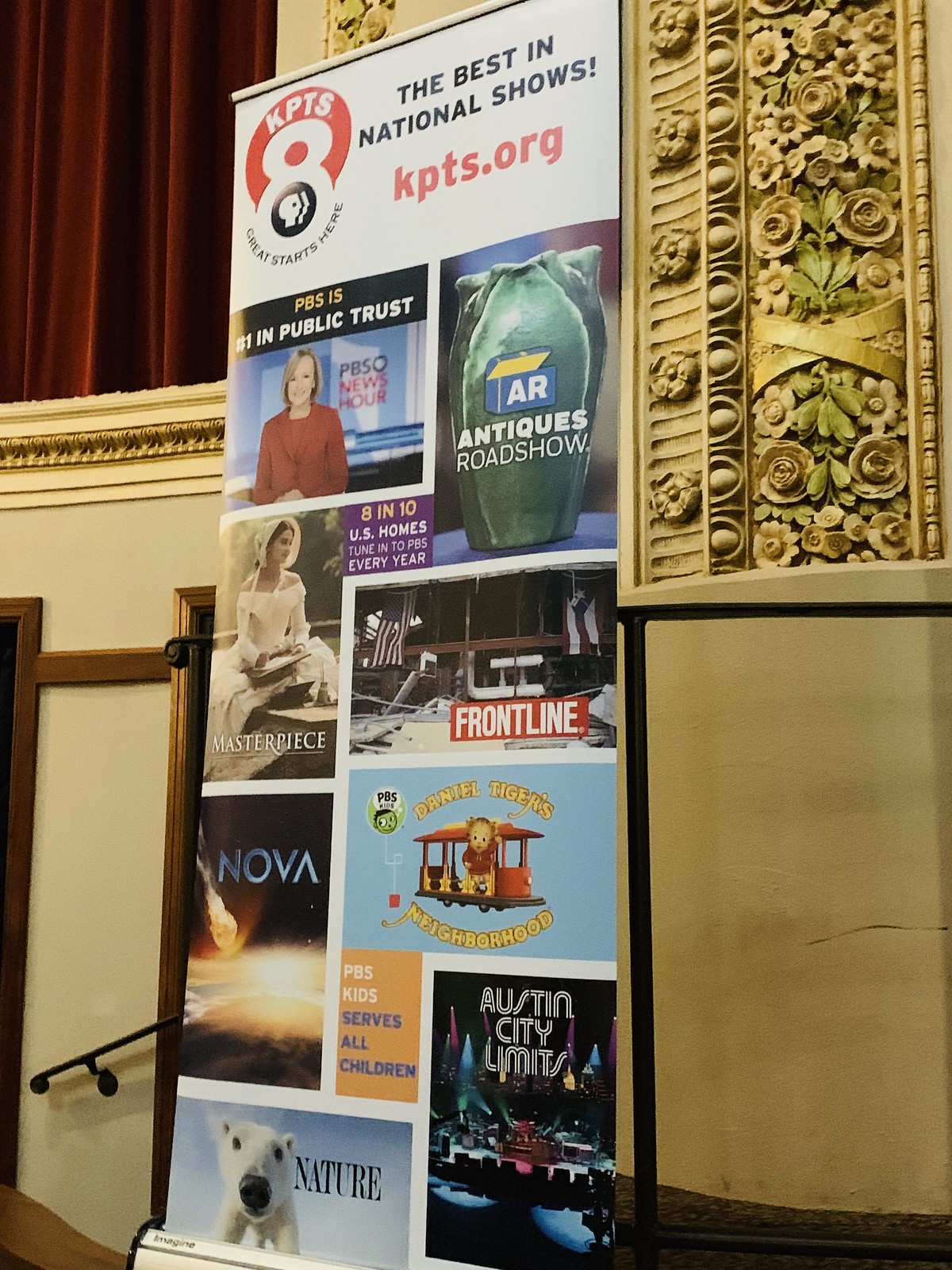The image depicts a large, ornate banner prominently positioned in what appears to be an elegant theater with intricate yellow walls adorned with gold floral designs and red stage curtains visible to the left. At the top of the banner, which has a white background, bold black text proclaims "The Best in National Shows" followed by "KPTS.org" in red. Just below, the KPTS logo, an orange background with a white "8" and "KPIS" in white, can be seen. The middle section of the banner features a collage of promotional images for various PBS shows. On the far left, "NOVA" is advertised with blue letters against a black background, suggesting a theme involving space. Next to it, "Antiques Roadshow" is highlighted above an artisan vase, while "Masterpiece Theater" displays an image of a woman in a red dress. "Frontline," positioned to the right, is another news program, and beneath it, "Daniel Tiger's Neighborhood," an animated children's show of a tiger character, emphasizes PBS's dedication to serving all children. To the far right, "Austin City Limits" is promoted alongside "Nature," showcasing a polar bear against a blue background. At the bottom of the banner, phrases like "PBS is number one in public trust" and "8 in 10 US homes tune in to PBS every year" are included, reinforcing the network's wide reach and trusted reputation. The banner itself appears set in front of an elegant column, adding to the overall sophisticated ambiance.